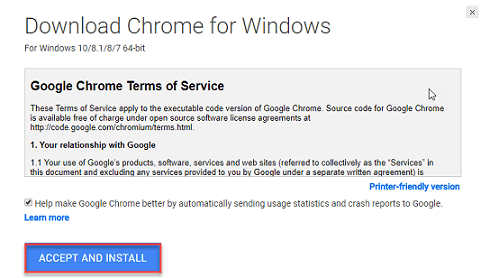The image features a prominently white background at the top, with the text "Download Chrome for Windows" displayed in large black letters. Just beneath it, in smaller black letters, it specifies "for Windows 10 / 8.1 / 7 / 8 / 7 64-bit."

A light gray box is positioned below this section, containing two main blocks of text. At the top of this box, in bold black letters, it reads "Google Chrome Terms of Service." Directly below, in smaller text, it states, "The Terms of Service apply to the executable code version of Google Chrome. Source code for Google Chrome is available free of charge under an open source software license agreement at http://code.google.com/chromium/terms.html."

Further down in the same light gray box, another paragraph begins with, "Your relationship with Google." It continues, "Your use of Google products, software, services, and websites, referred to collectively as the Services in this document, includes any services provided to you by Google under a separate written agreement."

Following this, a footer in the gray box reads, "Printer-friendly version. Help make Google Chrome better by automatically sending user statistics and crash reports to Google."

At the bottom of the image, a prominent blue rectangular button is featured, containing the text "Accept and Install" in white. This button is outlined by a red border on all four sides, making it stand out against the background.